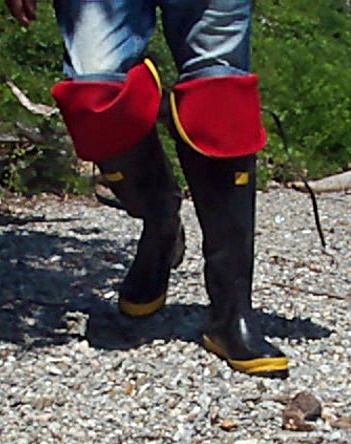This is a detailed close-up photograph of a person’s legs from the thighs down, captured outdoors. The background showcases vibrant, short green grass and a few trees, suggesting a natural setting. The individual is standing on rough concrete or gravel. They are clad in jeans, with tall black rubber boots that extend past the knee. The boots are distinctively designed with a red interior, folded down to reveal red fabric outlined in yellow at the knee. The boots feature a yellow square near the top by the calf and a yellow sole. The person's right foot is slightly ahead of the left one, which is raised, indicating movement as if they are walking forward. The shadow of the person and a glimpse of their hand can also be seen in the image. The attire and context suggest that the person may be engaged in an activity like hunting or fishing.